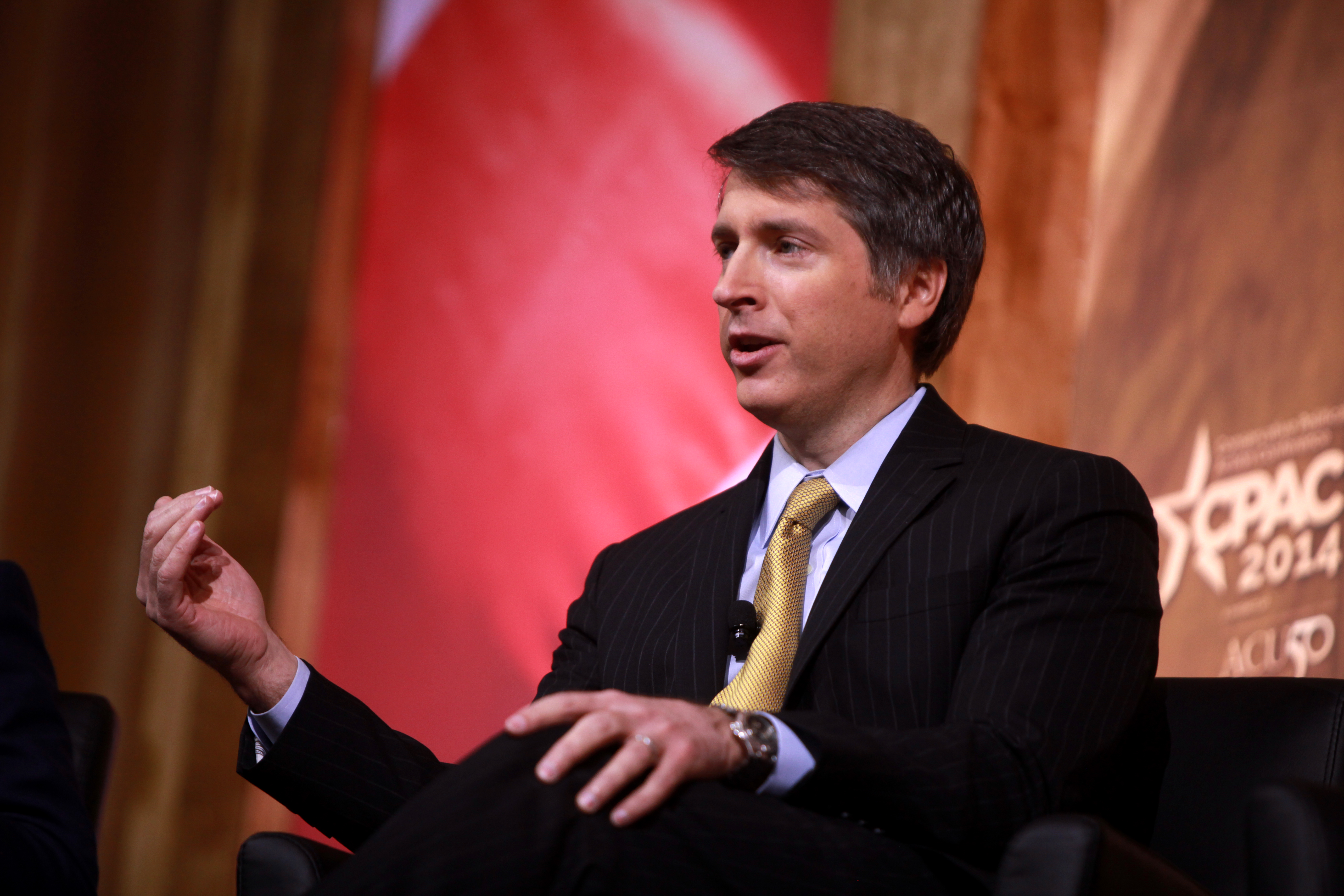In this image, a man is seated with one leg crossed over the other, raising his knee. He has dark, straight hair combed to one side, with distinguished streaks of gray near the temples, complementing his pointy nose. Captured mid-conversation, his mouth appears slightly open as if speaking. He is dressed in a black suit paired with a golden tie and a crisp white shirt. His hand rests on his knee, adorned with a watch and a ring, while the other hand is raised with his elbow bent, suggesting he is engaged in explaining something. The backdrop features an arrangement of red, brown, and white lights, casting vibrant streaks that enhance the scene's dynamic feel. The setting hints at a stage environment likely shared with other individuals, indicated by the diffused figures in the background.